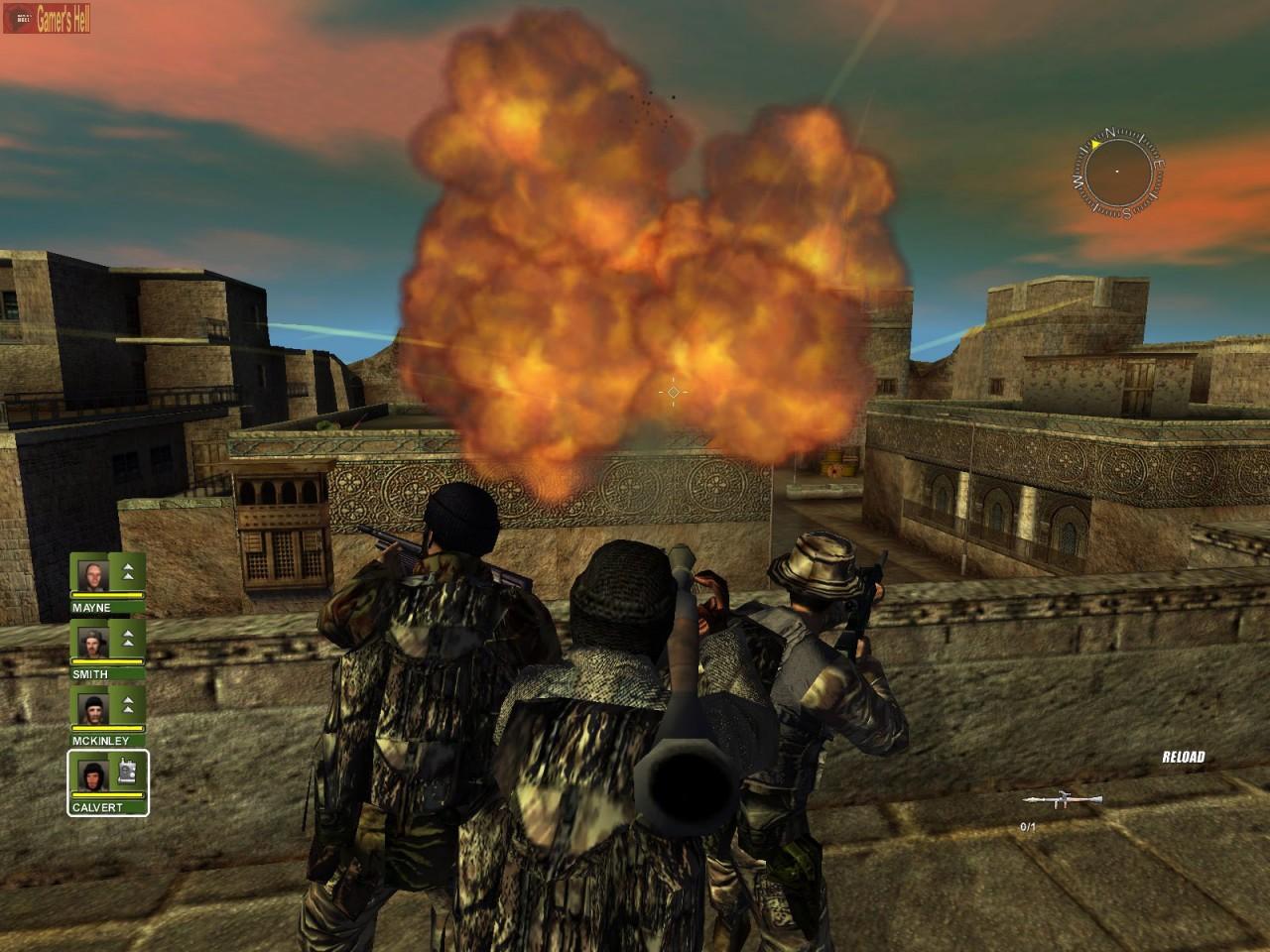This image is a dynamic screenshot from a computer or video game, prominently featuring an action-packed scene. Superimposed on the image are infographics comprising small green squares arranged vertically, each containing a photograph that likely represents computer game players.

In the foreground, three characters clad in army-style attire stand poised with guns and various weapons, exuding a rugged, perhaps Native American-inspired aesthetic. They are situated within a distinctive architectural environment characterized by square-shaped, stone buildings adorned with intricate mosaic patterns. Dominating the center of this urban landscape is a massive fireball explosion, infusing the scene with intense drama and energy.